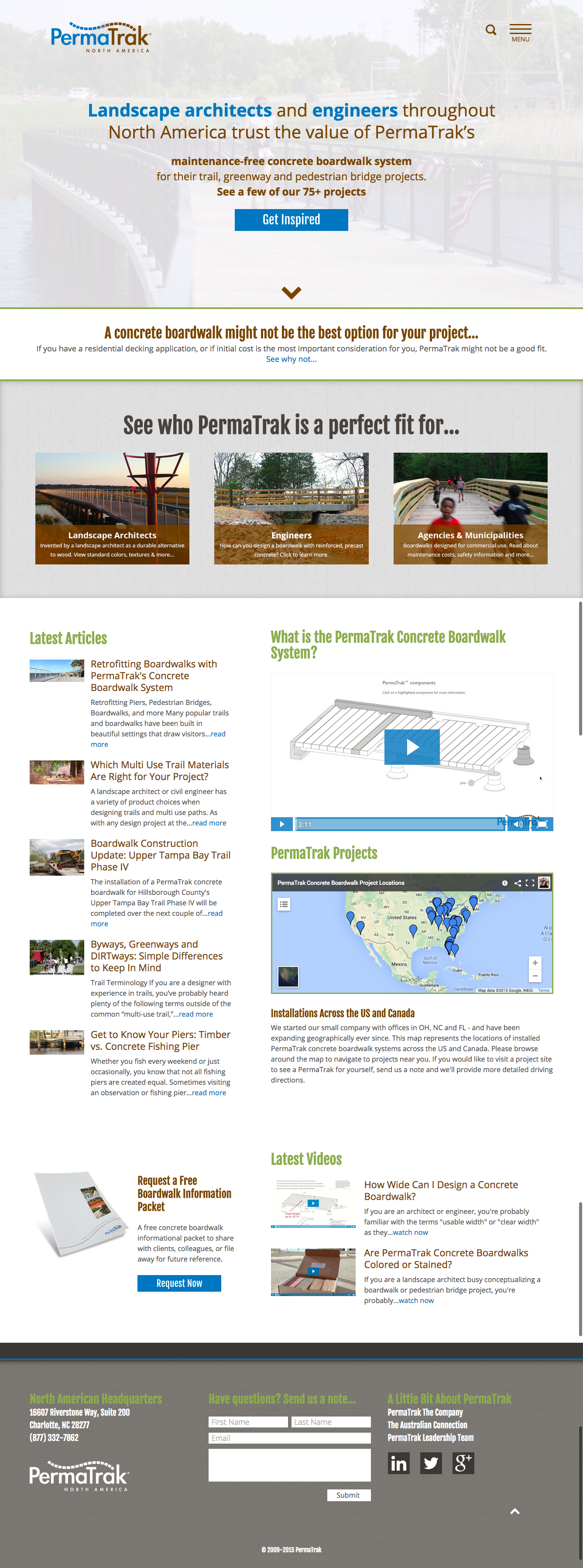This image is a screenshot of a webpage viewed on a smartphone. The layout is vertical, with the top section featuring the title "Permatrack, North America" in blue and brown text, placed within a rectangular banner displaying a filtered image background. The background image appears to depict a bridge spanning over water with trees in the vicinity.

Beneath the title, in blue and brown text, it states: "Landscape architects and engineers throughout North America trust the value of Permatrack's maintenance-free concrete boardwalk system for their trail, greenway, and pedestrian bridge projects. See a few of our 75-plus projects." A blue button labeled "Get Inspired" is prominently displayed for user interaction.

Further down, the webpage presents a light gray rectangle with the text, "See who Permatrack is a perfect fit for," followed by three labeled images:
1. "Landscape Architects" showcasing a bridge.
2. "Engineers" featuring another type of bridge.
3. "Agencies and Municipalities" depicting a crowd of people walking over a bridge.

The lower portion of the screenshot contains a white background filled with text and a map of North America marked with several pins, indicating project locations. This section explains the creation process of the Permatrack concrete boardwalk.

Additionally, there are embedded videos accessible at the bottom, accompanied by the company's contact information, including the address and other relevant details.